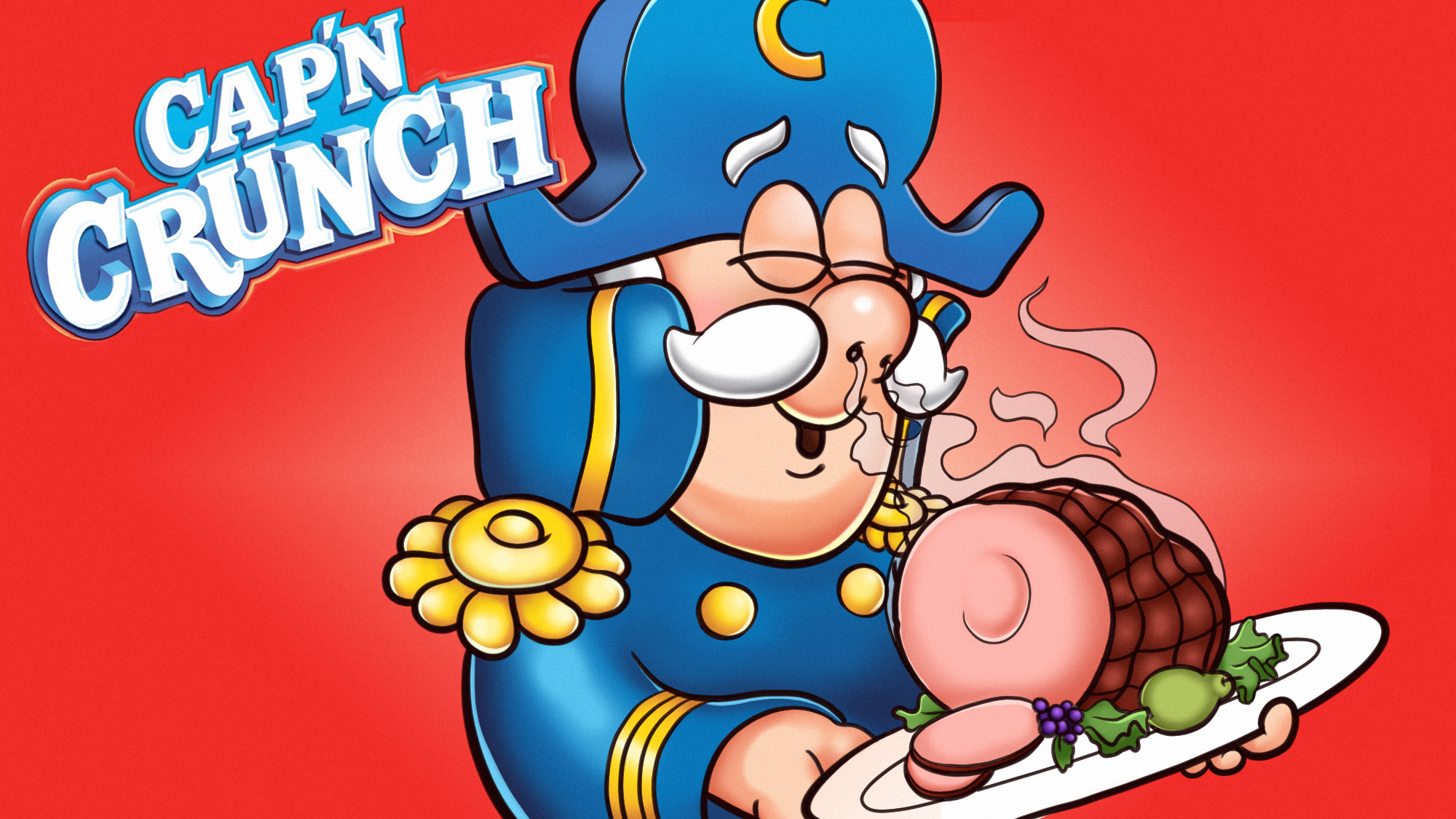This rectangular, hand-drawn cartoon image depicts the iconic Captain Crunch in his recognizable sailor outfit. The background features a vibrant red and white gradient, with the words "CAP'N CRUNCH" prominently displayed in white, all-caps letters against a blue backdrop in the top left corner. The captain himself, characterized by his white mustache and white hair, is wearing his signature blue uniform adorned with yellow buttons, emblems, and sleeve markings, as well as a blue captain's hat marked with a yellow "C."

The captain stands holding a plate of freshly cut ham, with a couple of slices at the edge, complemented by green lettuce leaves, and what appear to be blueberries or grapes. Steam, illustrated as white wisps, emanates from the ham, curling up towards the captain's nostrils. Captain Crunch's eyes are closed, and he displays a broad smile, clearly savoring the aroma of the freshly cooked ham. The detailed artwork captures the essence of the beloved cereal mascot enjoying a delightful, sensory moment.